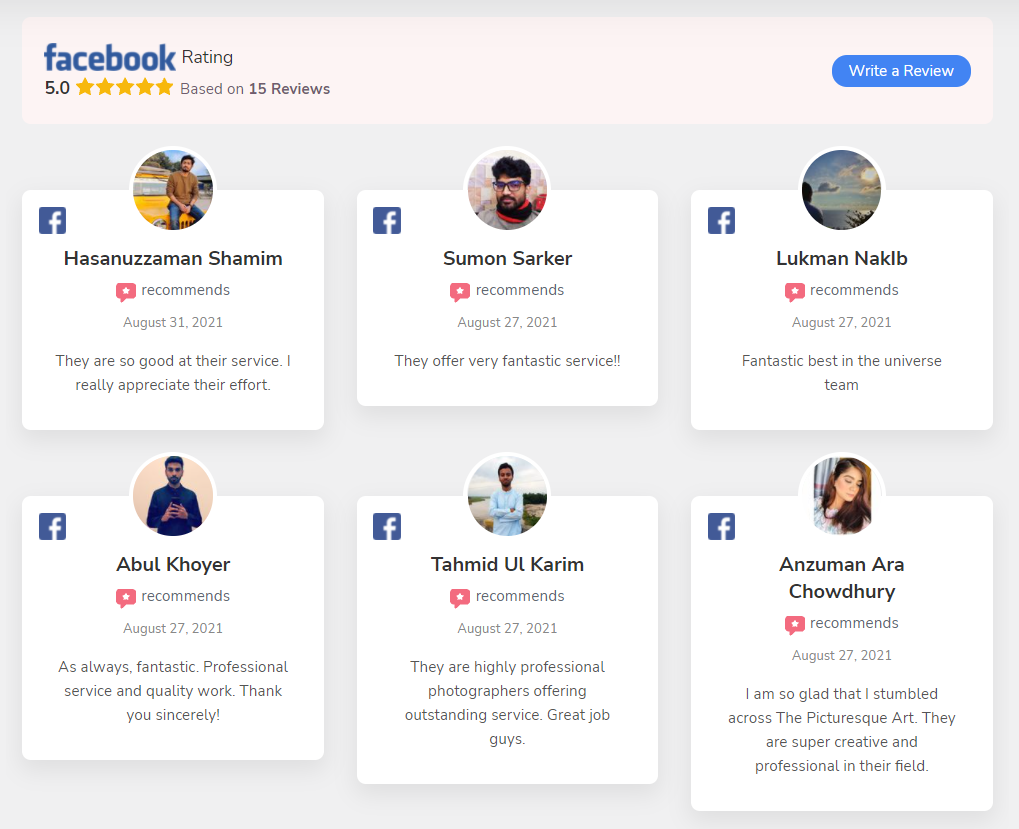**Caption:** *(Facebook Reviews Screenshot)*

This screenshot captures a positive Facebook rating for a service, boasting a perfect score of 5 stars out of 5, based on 15 reviews. At the top of the screenshot, the iconic Facebook logo is displayed in lowercase, bold, blue letters, with the word "rating" in smaller, plain black text. To the right, a blue, rounded rectangle features the prompt "Write a review" in white writing.

The image showcases six favorable reviews, all dated August 27th, 2021, from different users. The reviews are as follows:

1. **Hasanuzaman Shim** - "They are so good at their service, I really appreciate their effort."
2. **Suman Sarkar** - "They offer very fantastic service."
3. **Lukman Nakib** - "Fantastic, best in the universe team."

On the second row:

4. **Abdul Koya** - "As always, fantastic, professional service and quality work, thank you sincerely."
5. **Tamid Al Karim** - "They are highly professional photographers, offering outstanding service. Great job, guys."
6. **Anzuman Ara Chowdhury** - "I am so glad I stumbled across the picturesque art. They are super creative and professional in their field."

While it's slightly suspicious that all six reviews are dated the same day, the service maintains a stellar rating with consistent positive feedback.